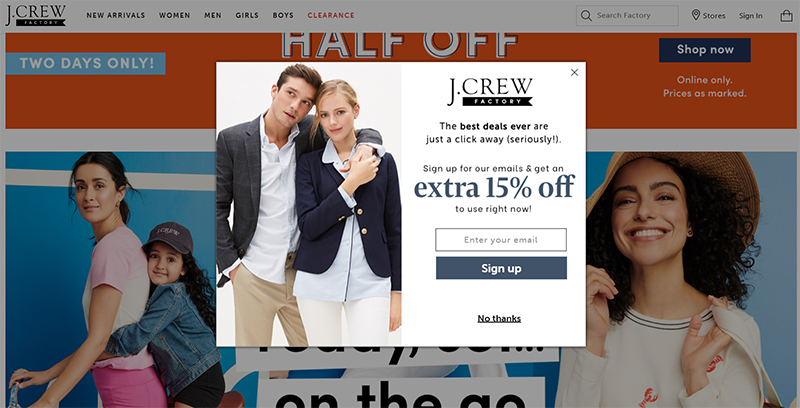The image depicts a J.Crew Factory website homepage featuring a central pop-up window. The popup, which has a white background, showcases two models—a boy and a girl. The text in the popup reads: "J.Crew Factory: The best deals ever are just a click away (seriously!). Sign up for our email to get an extra 15% off to use right now." It includes a field for entering an email address, a "Sign Up" button, and a "No Thanks" option.

Above the popup, the website's banner is visible, including the J.Crew logo and navigational links to "New Arrivals," "Women," "Men," "Girls," "Boys," and "Clearance" (with "Clearance" highlighted in orange). On the right side, there is a search icon labeled "Search Factory," an icon for store locations, a "Sign In" link, and a shopping bag icon.

Below the banner, an orange promo bar states "Half Off," and adjacent to it, a blue banner reads "Two Days Only!" with white text. To the right, a navy blue square with white text says "Shop Now." Beneath this promotional section, smaller white text states "Online Only Prices as Marked." The lower part of the image shows various models displaying different clothing items available on the website.